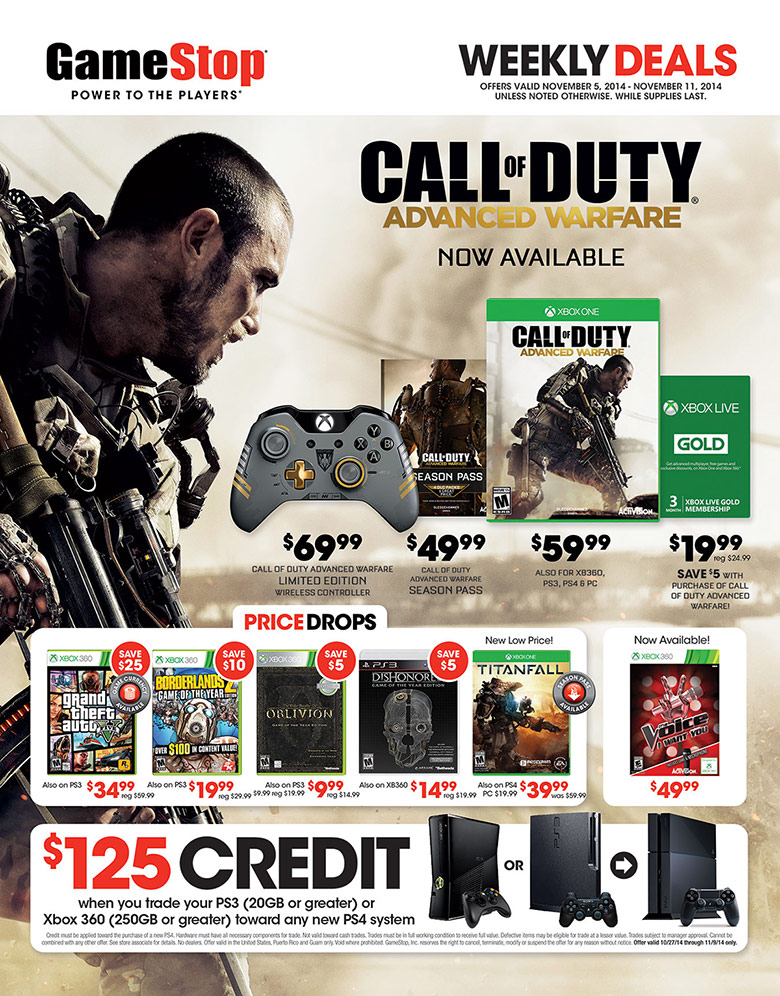Screenshot of a GameStop advertisement showcasing weekly deals valid from November 5th, 2014, to November 11th, 2014, while supplies last. The official GameStop logo is prominently displayed in the top-left corner, with "GameStop" in black and red text, followed by the slogan "Power to the Players." On the right, the ad highlights the release of "Call of Duty: Advanced Warfare," featuring various related offers. The advertisement features an image of a sleek grey, black, and gold controller priced at $69.99, a season pass for $49.99, and the game itself for $59.99. Additionally, an Xbox Live Gold membership is available for $19.99.

Below this section, the ad lists notable price drops on several games, including "Grand Theft Auto V," "Borderlands 2," "Oblivion," "Dishonored," "Titanfall," and "The Voice." Finally, there is a mention of a $125 credit available for trading in gaming consoles.